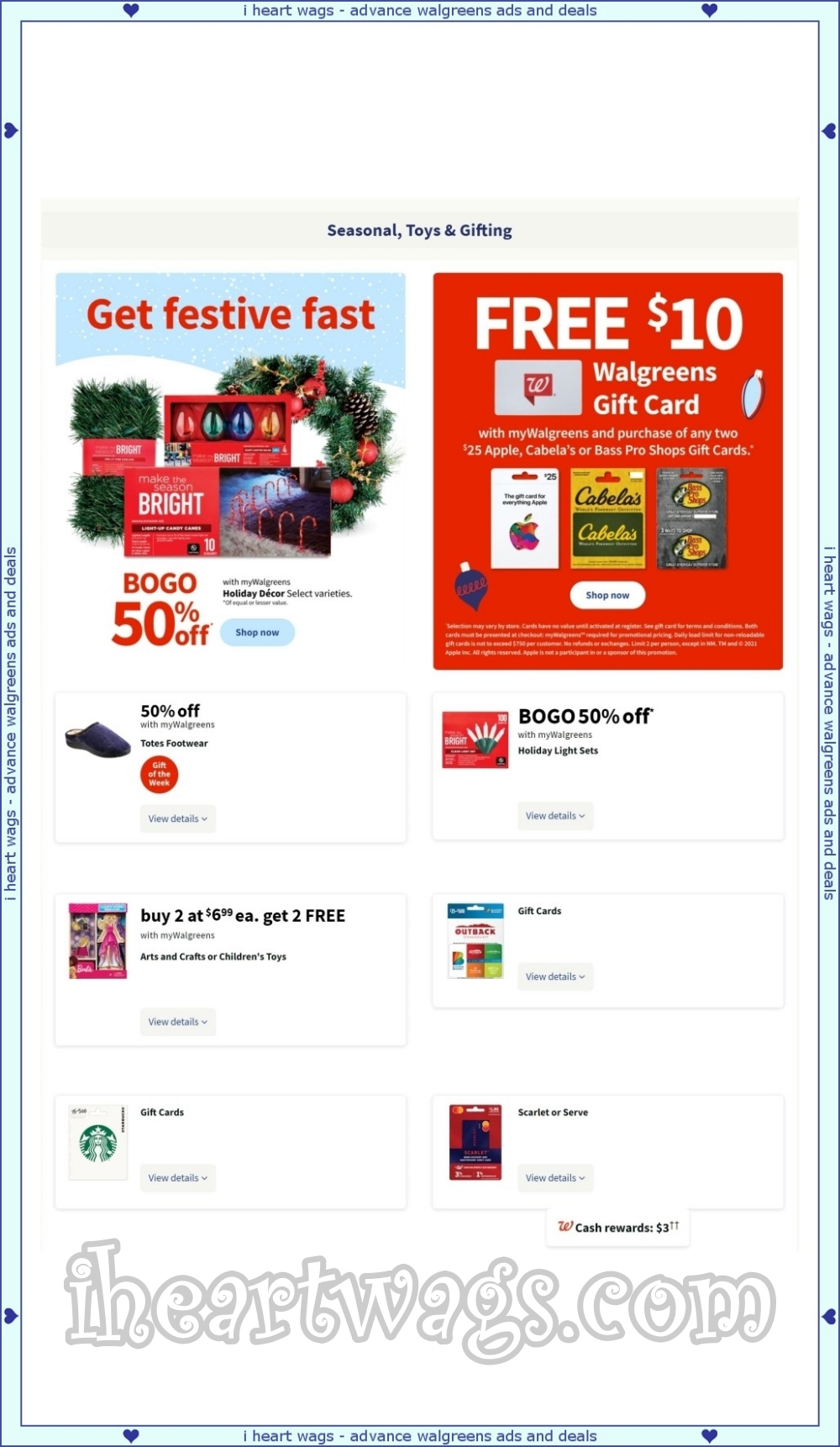In this detailed advertisement image, we see a neatly organized layout divided into various sections, bordered by a light blue rectangular frame. 

At the top, the image features a white background with a clean transition to a light gray background displaying the text "Seasonal Toys and Gifting" in bold black letters.

To the left side of the image, a vibrant section urges viewers to "Get Festive Fast" in striking red text. Accompanying this cheerful message are images of festive wreaths and various Christmas-related items. A prominent "BOGO 50% off" offer in red text sweetens the deal for holiday shoppers.

On the right, a bold red square stands out with the enticing offer of a "Free $10 Walgreens Gift Card" advertised in large white font. Below this, there are three gift cards neatly arranged: the first being white, the middle one in yellow and black, and the rightmost in gray and gold. The small white sentences provide additional details, though they are not clearly legible.

Continuing below on the left section, another offer boasts "50% off" on a pair of black shoes, while the right reiterates the "BOGO 50% off" deal. Moving further down, a promotional offer is displayed mentioning "Buy Two" items, although it's difficult to identify the exact product due to the zoomed-out nature of the image. There's a white and blue package nearby, adding to the showcase.

Towards the bottom, a recognizable Starbucks gift card is featured prominently. To the right is a visually striking red and black image. Concluding the advertisement at the very bottom, the website "Iheartwags.com" is displayed in a unique font where the letters are white on the inside and outlined in gray.

This intricate and vibrant advertisement effectively catches the eye with its array of festive and promotional offers, meticulously organized for a clear and engaging presentation.